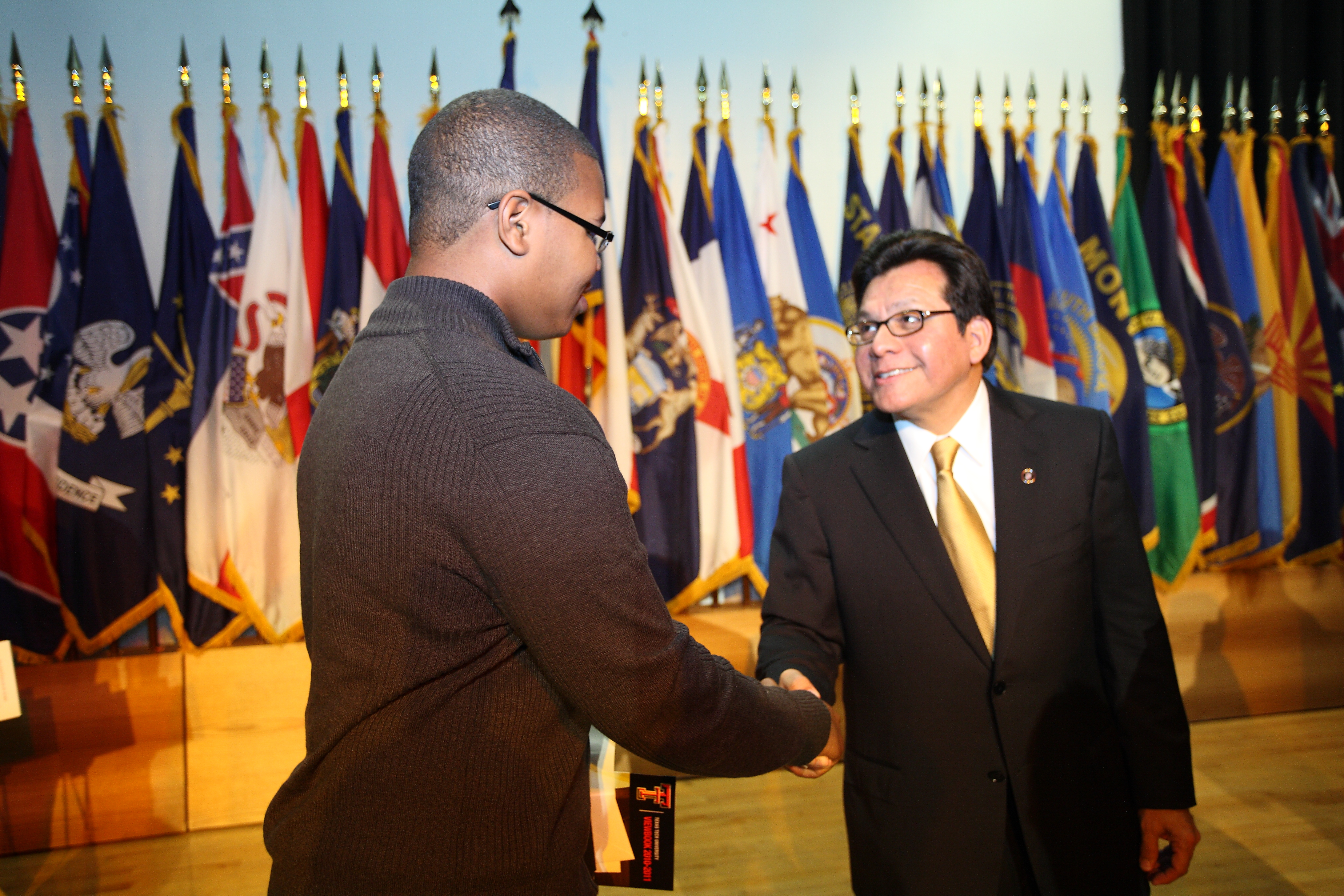This photograph captures a moment of camaraderie between two men shaking hands on what appears to be a wooden stage with a blue backdrop, possibly at the United Nations given the array of diverse flags in the background. On the left is a younger African American man, likely in his late teens or early twenties, with short brown hair and black-framed glasses. He's dressed in a brown sweater. On the right stands an older Caucasian man, recognizable as a politician, wearing a black suit jacket adorned with a pin, a gold tie, and a white collared shirt. Both individuals are smiling warmly at each other, exuding a sense of mutual respect. The flags behind them, with colors ranging from navy and royal blue to red, white, kelly green, and gold, add to the international and formal ambiance of the setting.